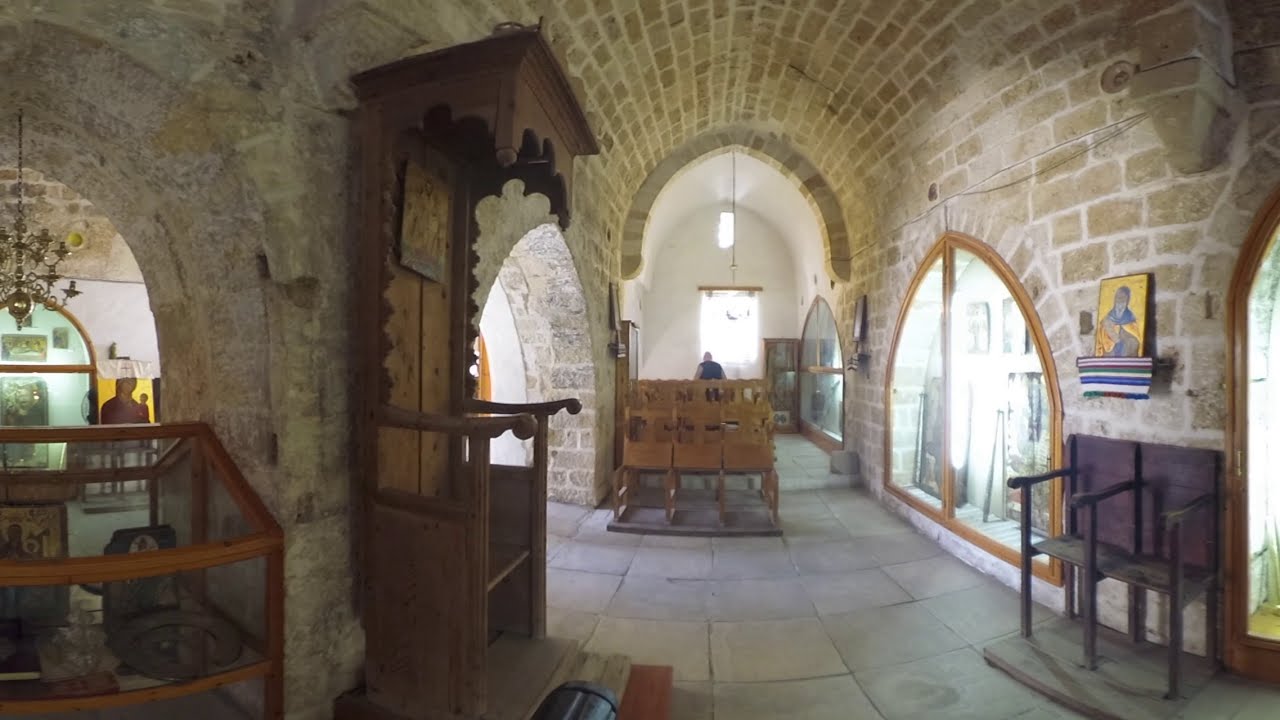Inside this historic, likely 19th-century church, the old-world architecture is beautifully captured. The photo reveals a charming, brick-lined interior with several graceful arches. The stone slab flooring complements the numerous wooden furniture pieces dotted around. On the left side of the image, there is a prominent, large wooden bench featuring an intricately carved hood, stained to highlight its ornate design. Nearby, simple, plain wooden chairs sit together. The center of the frame is dominated by an archway leading the eye towards the back of the room, where sunlight filters through a window or an opening. To the right, a glass display cabinet stands with a distinctive spearhead shape, accompanied by three more ornate wooden chairs below a golden-blue portrait of a saint. Another glass cabinet is tucked in the back left corner. A figure, possibly a church attendant or preacher, is visible near the window, adding a touch of human activity to the serene atmosphere. Above, the ceiling is striking with large square stones lining its descent. The scene evokes a calm, timeless aura, enhanced by the sunlight streaming in and hinting at the building's long, storied past.